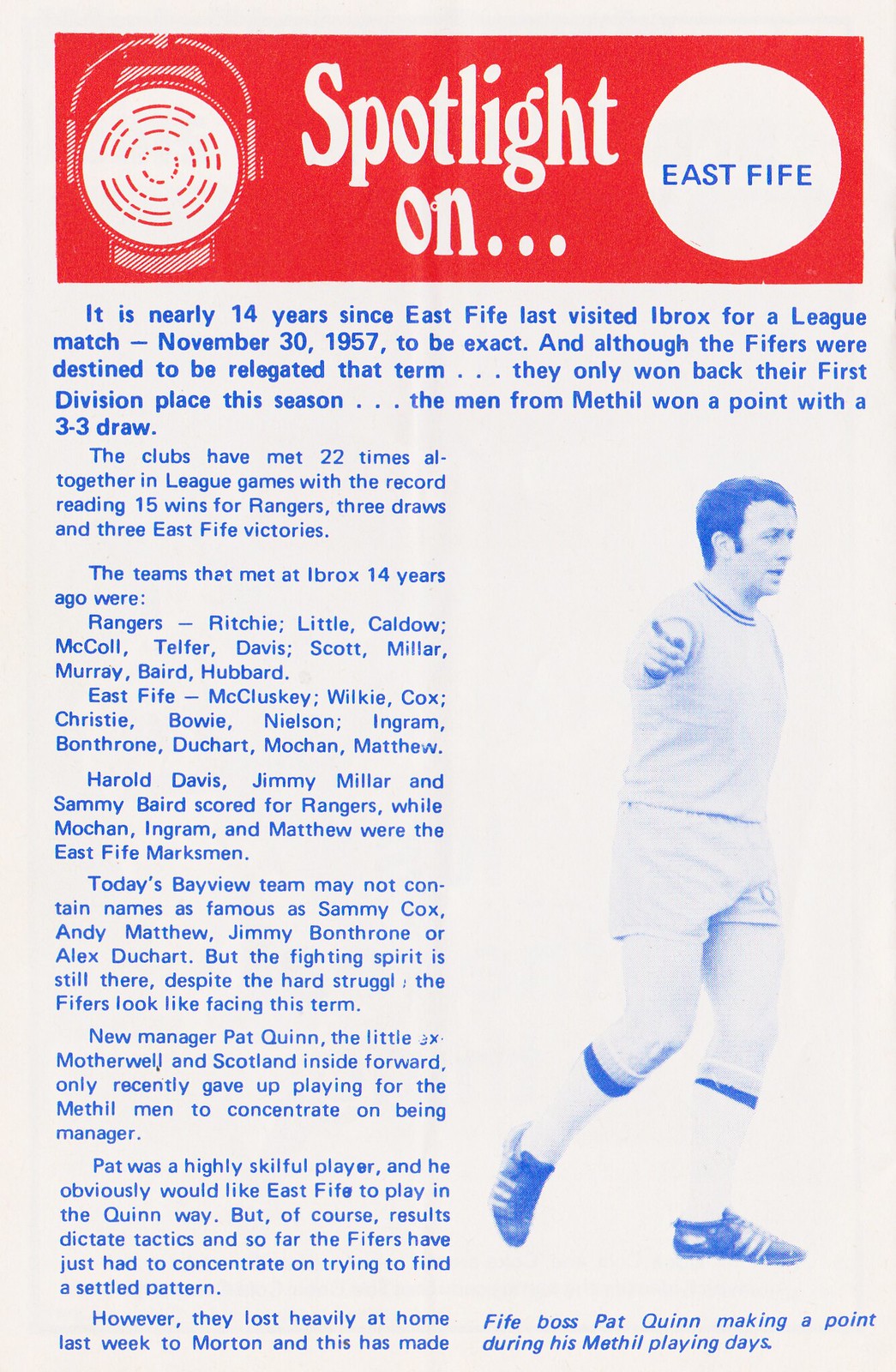The image is a rectangular poster resembling a page from a Soccer Magazine, set against an off-white background similar to newspaper print. Dominating the top portion is a thick red horizontal strip, taking up about one-fifth of the poster, with the words "SPOTLIGHT ON" prominently displayed in white lettering, accompanied by an illustration of a spotlight on the left. On the right of the red strip, there's a white circular icon with "East Fife" written in blue. Below this header, the main article appears in blue text, consisting of 6 to 8 paragraphs detailing the historical performance and current state of the East Fife soccer team. Notably, it recounts their league matches against Rangers, highlighting specific games and key players from both teams, including the draw on November 30, 1957. The right side of the poster features a blue and white image of Pat Quinn, East Fife's manager, in a full-body shot pointing towards the viewer. Below the picture, a caption reads, "Fife boss Pat Quinn making a point during his Methill playing days."